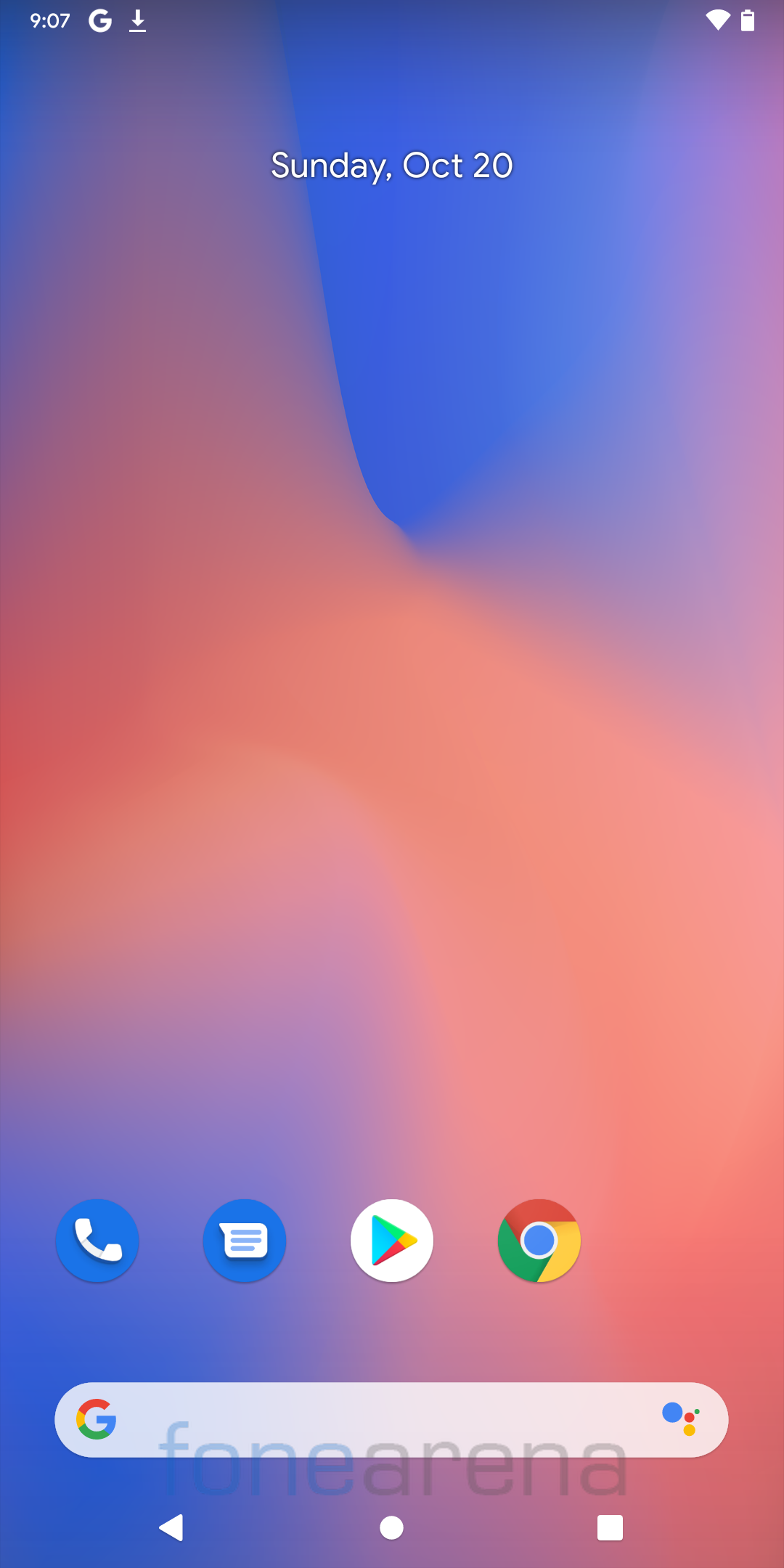Here's the cleaned-up and detailed descriptive caption:

This screenshot features the interface of a mobile phone application with an artistic background depicting a salmon pink hourglass, rotated 45 degrees, set against a bright blue, hazy backdrop. At the top center, white text indicates the date: "Sunday, October 20." The bottom of the screen displays four icons. From left to right: a blue circle with a white phone icon, a blue circle with a white chat box featuring light blue lines, a white circle adorned with a multicolored, right-pointing triangle, and a multicolored circle divided into a green bottom-left section, a red top section, and a yellow bottom-right section. In the center is a blue circle surrounded by a white outline. Below these icons lies a white search bar. On the left of the search bar is a multicolored "G" icon, and on the right is a cluster of multicolored circles comprising a central red circle, a small green circle in the top right, a medium-sized yellow circle at the bottom, and a large blue circle at the top left. A translucent watermark reading "Phone Arena" spans across the bottom of the search bar and the underlying background. Finally, three navigation icons are situated at the very bottom of the screen: a white left-pointing triangle on the left, a white circle in the middle, and a white square with rounded corners on the right.